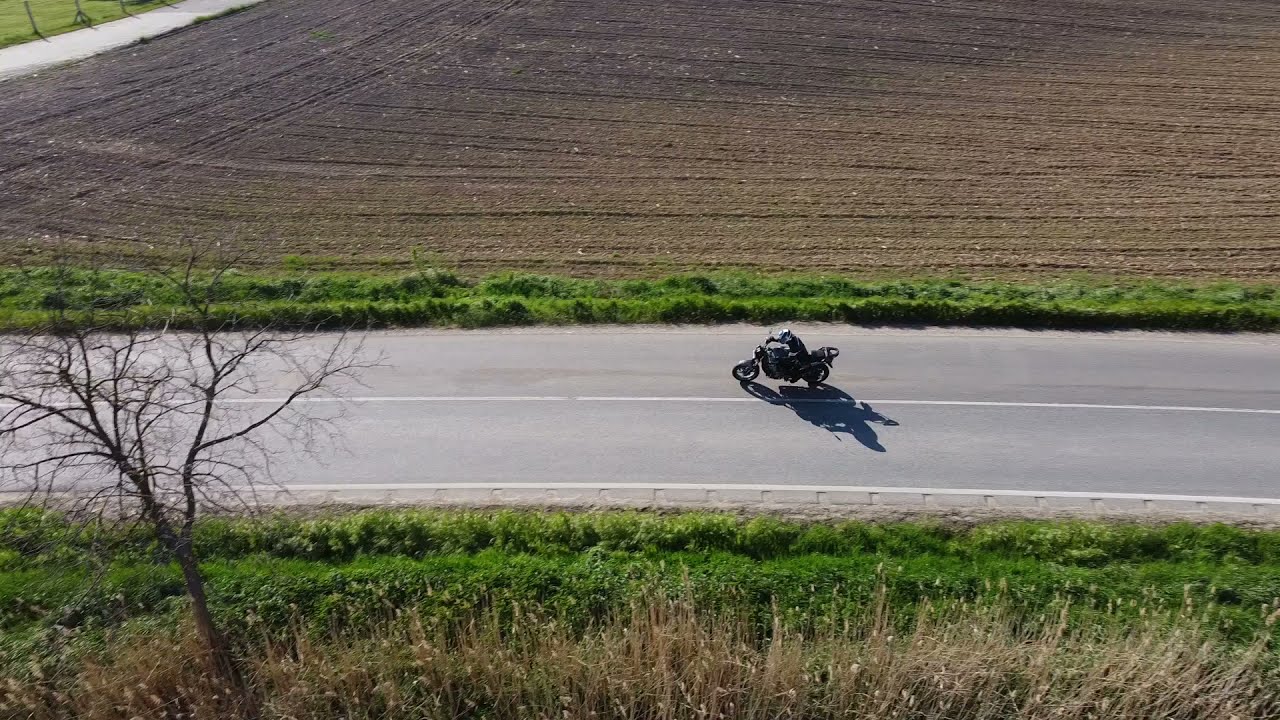The image depicts a lone motorcyclist, dressed in black protective gear and a helmet, riding a black motorcycle on a two-lane, gray, concrete road that runs horizontally across the center of the frame. The road features a single white stripe dividing the lanes. On either side of the road lies greenery, marked by rows of gray rectangular bricks at the close edge, giving way to light brown shrubbery and grass, appearing somewhat wheat-like at the bottom of the image. In the far background, a large, freshly plowed field with geometric, striated lines of light brown soil stretches across the horizon, bordered by a small road at the top left corner. The image also includes a tree with no leaves situated in the bottom left corner, casting a shadow towards the lower right corner. The entire scene is devoid of any other traffic, emphasizing the solitary journey of the motorcyclist.